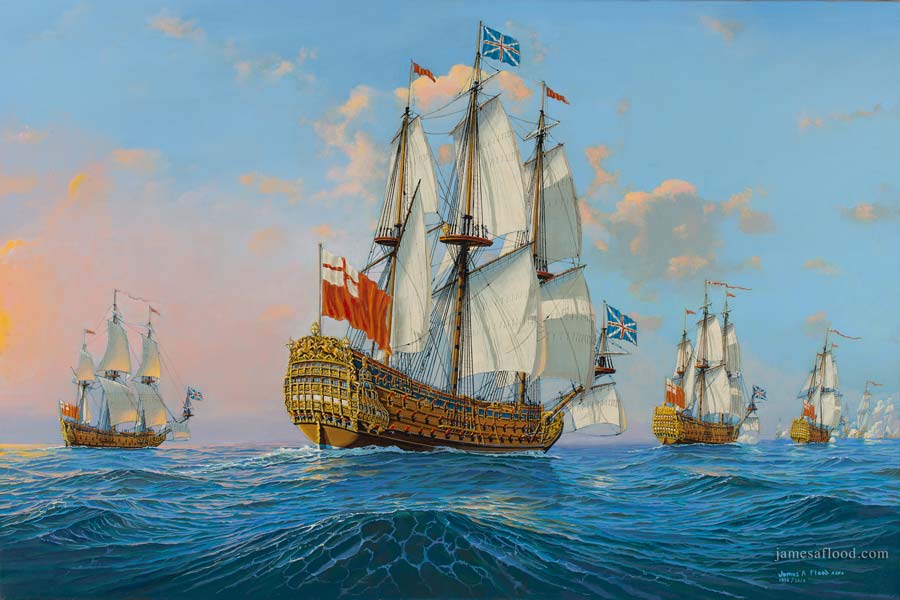This artwork, set in a horizontally aligned rectangle, captures a fleet of vintage sailboats navigating choppy blue waters. The centerpiece is a grand sailboat with a brown wooden hull and six large white sails distributed across three masts. The tallest mast prominently displays a British flag, while red flags adorn the two smaller masts. Another British flag hangs at the back of the ship, and the front of the vessel features a large red flag with an orange cross against a white background. Additional sailboats, identical in design and adorned with similar flags, are visible behind the central boat to the right, with a single boat to the left. The sea beneath wraps in waves, featuring white-tipped crests. Above, the sky is mostly clear with feathery white and gray clouds, and an area of pale orange clouds in the middle-left section. The detailed painting includes the artist's watermark, "jamesaflood.com," in white print in the lower right corner, reinforcing its authenticity.